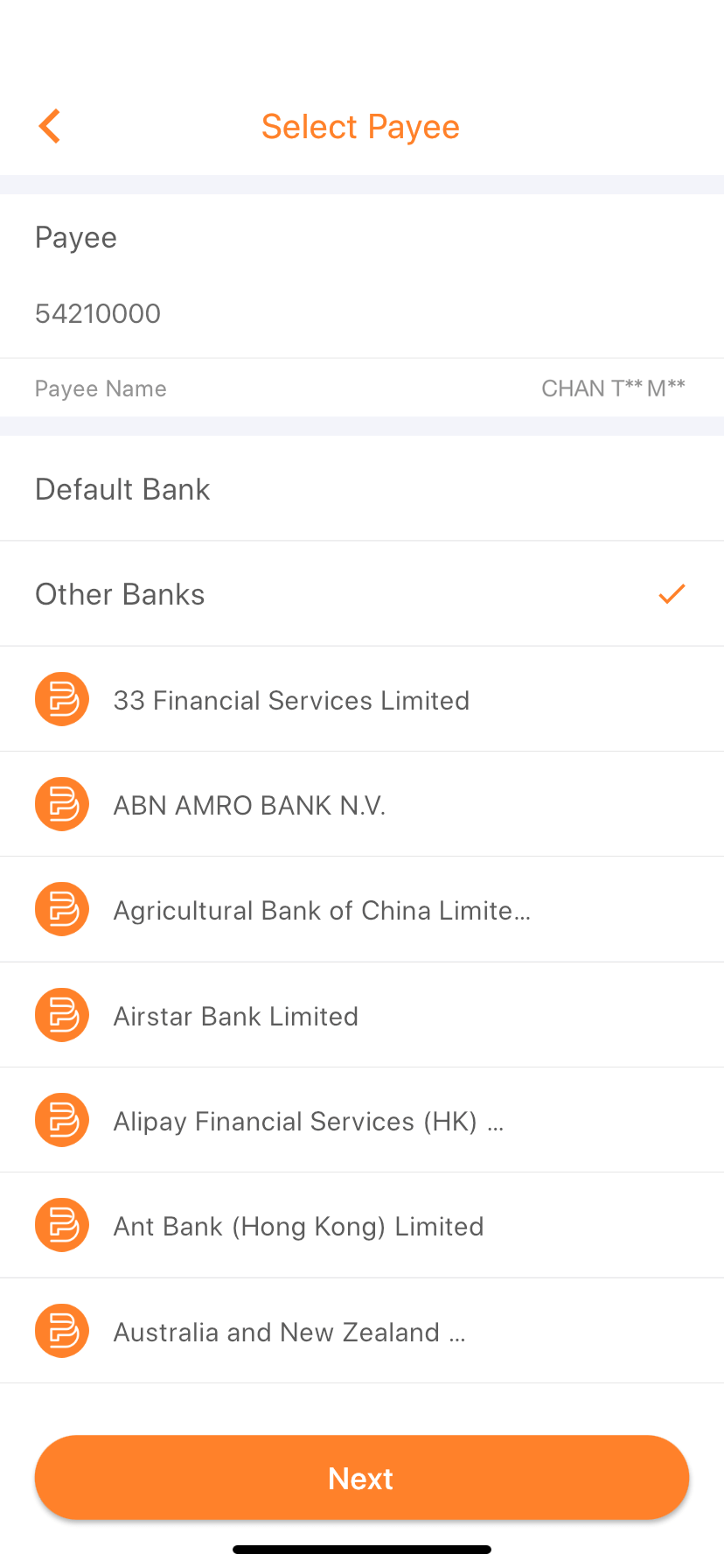This image captures a screenshot from a cellphone displaying a digital interface for selecting a payee. At the top of the screen, there is an orange-colored header with the text "Select Payee" and a left-pointing arrow. Below this header, a thin gray line acts as a separator.

The next section is titled "Payee," featuring the detail "542100000" directly underneath it. Following this is the "Payee Name," which reads "CHANT" with hyphens and an "M" afterward. A labeled section for "Default Bank" is present, but specific details are obscured. There is also a category for "Other Banks," which ends with an orange checkmark.

Seven distinct areas follow, each marked with an orange circle containing white squiggly lines, signifying different entities or countries:

1. "33 Financial Services Limited ABN"
2. "Bank NB"
3. "Agricultural Bank of China Limited"
4. "Airstar Bank Limited"
5. "Alipay Financial Services HKEY"
6. "Ant Bank Hong Kong"
7. "Australia and New Zealand"

At the bottom of the screen, there is an orange "Next" button.